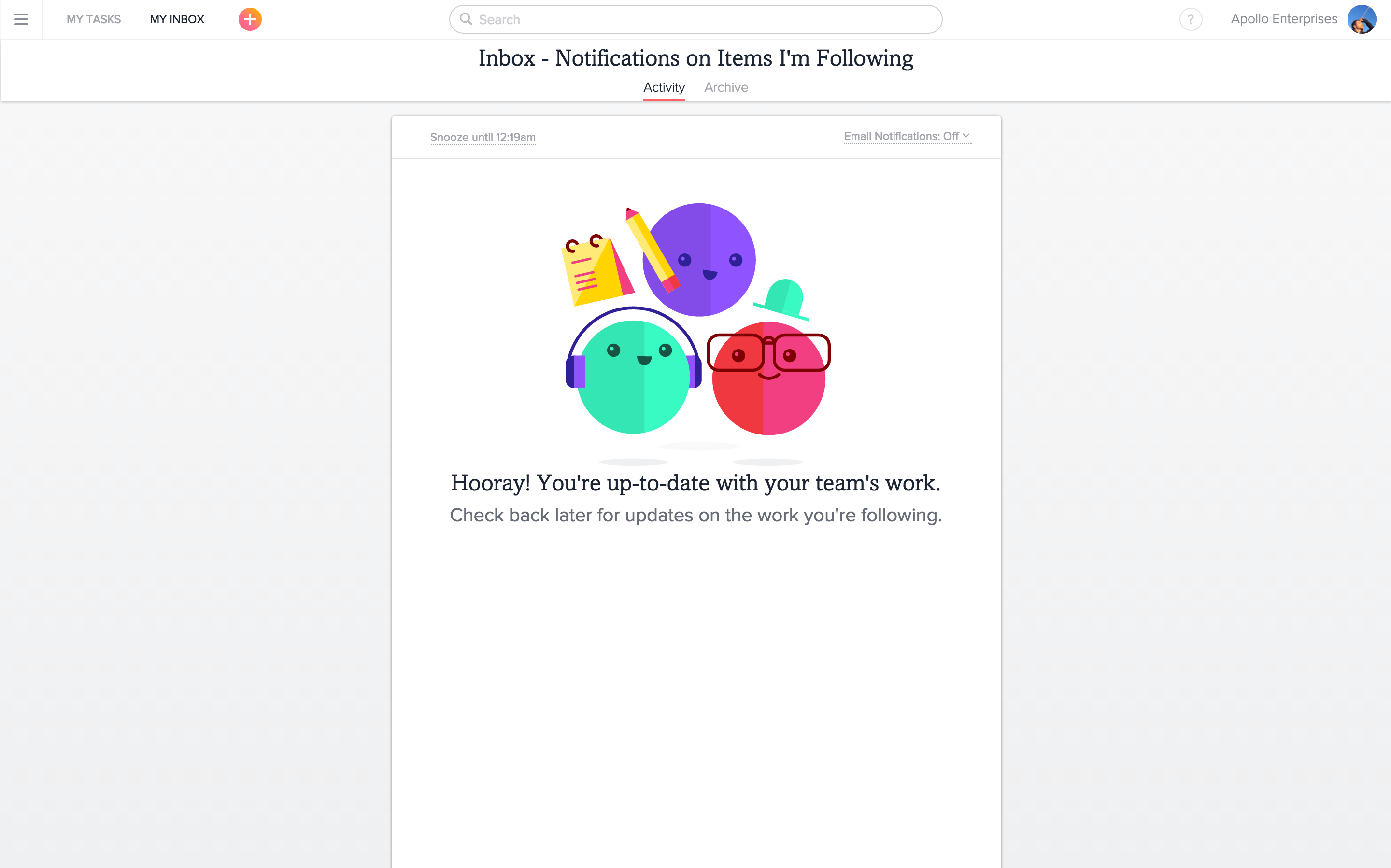The image features a user interface set against a pale purple background. At the top, there is a white rectangular box containing three small horizontal lines, followed by the titles "My Tasks" and "My Inbox." Nearby, a small red circle with a white plus sign is visible, alongside a search button. Adjacent to these elements, there is a user’s name accompanied by a round profile picture.

Directly below, the text "Inbox Notifications on Items I’m Following" appears, with the word "Activity" highlighted in red beneath it. A small white drop-down box is present, containing various icons and characters. 

First, there is a small yellow tablet icon. Adjacent to it, a purple circle features a face with a pencil beside it. Following that, a blue circle shows a face wearing purple headphones. Additionally, a pink and red circle displays a face wearing glasses and a blue hat.

At the bottom of the interface, the text reads, "Hooray! You're up-to-date with your team's work. Check back later for updates on the work you're following."